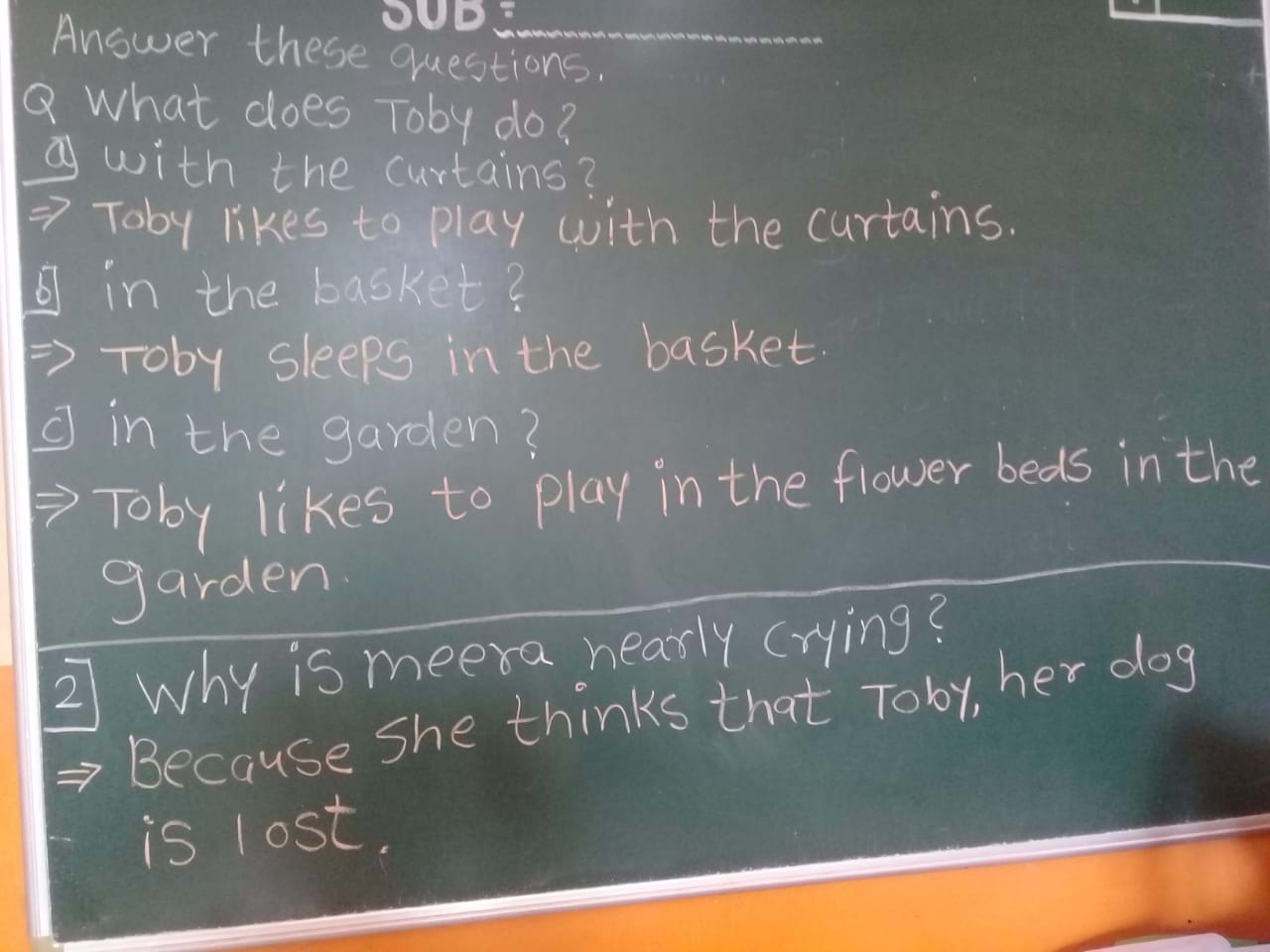In the image, a large green chalkboard dominates the scene, filling almost the entire frame. The chalkboard is positioned centrally against an orange wall that is visible around its edges on the bottom, left, and right sides. The setting seems to be a classroom, likely indoors during the day. On the chalkboard, written in chalk, there are several questions and answers in handwriting. The text reads: "Sub, answer these questions. What does Toby do with the curtains? Toby likes to play with the curtains. In the basket, Toby sleeps in the basket. In the garden, Toby likes to play in the flower beds in the garden. Why is Mira nearly crying? Because she thinks that Toby, her dog, is lost." The color palette of the image includes orange, white, green, gray, and tan, contributing to a warm and educational atmosphere.